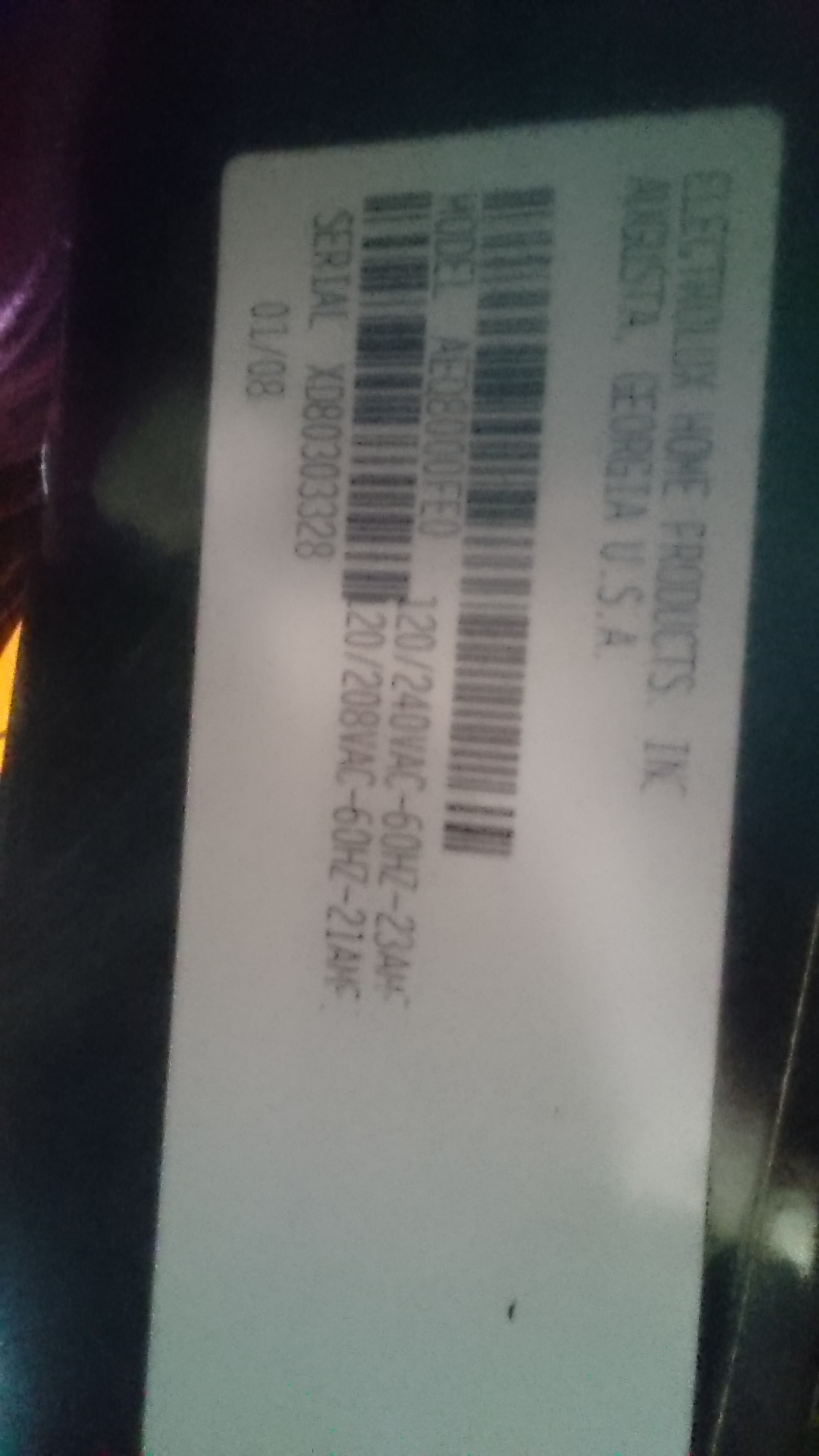This is a dark, blurry photograph of a white rectangular barcode label affixed to a shiny black surface, oriented with the left corner at the top and the right corner aimed towards the bottom. The top of the label reads "Electrolux Home Products, Inc., Augusta, Georgia, USA" in faded black font. Below this heading, there is a long barcode followed by a model number that reads "AE08000FE0." Beneath the model number, another shorter barcode is visible, approximately half the length of the first. This barcode is accompanied by detailed specifications: "120/240 VAC - 60 Hertz - 24 M AMF." Further down, a serial code number can be seen along with "01/08" at the very bottom of the label. Additionally, to the side of the lower barcode, a series of stacked product code numbers made up of letters and numbers is observed. The photograph also captures a light source reflection towards the bottom right corner.